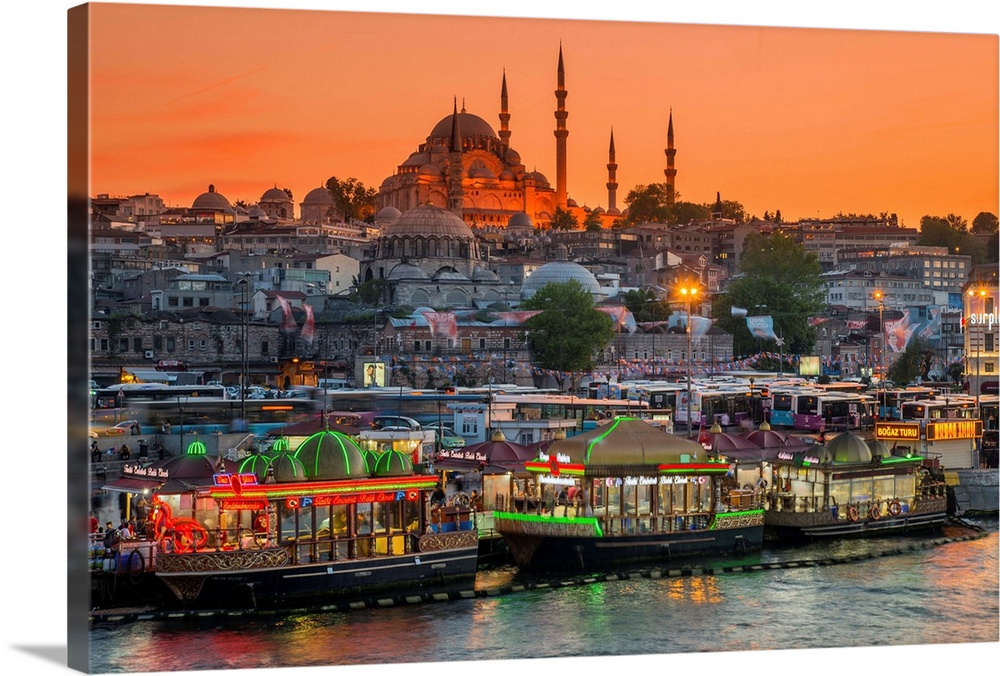The image depicted is a vibrant and realistic canvas painting of a large, historic city that resembles Istanbul. The bottom eighth of the image features a serene body of water reflecting the vivid neon lights from several docked houseboats, which appear to function as restaurants. The boats bear the text "Bogaz," adding to the impression of a bustling waterfront. Just above the water, a row of these illuminated houseboats spans the scene from left to right. 

In the middle third of the image, the city’s diverse architecture is showcased, with numerous buildings, including several with dome-shaped roofs. One particularly prominent, dome-topped structure, slightly offset to the top center-left, seems to be a historic landmark, potentially a well-known temple or mosque, and is surrounded by large spires. This building, glowing with an orange light, becomes a focal point against the dense urban backdrop. 

The top fourth of the painting captures a stunning sunset sky, blending hues of yellow, pink, and orange, further enhancing the dynamic ambiance of the cityscape. The trees intermingle with the urban structures, and the entire scene is bathed in a warm, inviting light that highlights the clear and vibrant details of the city.